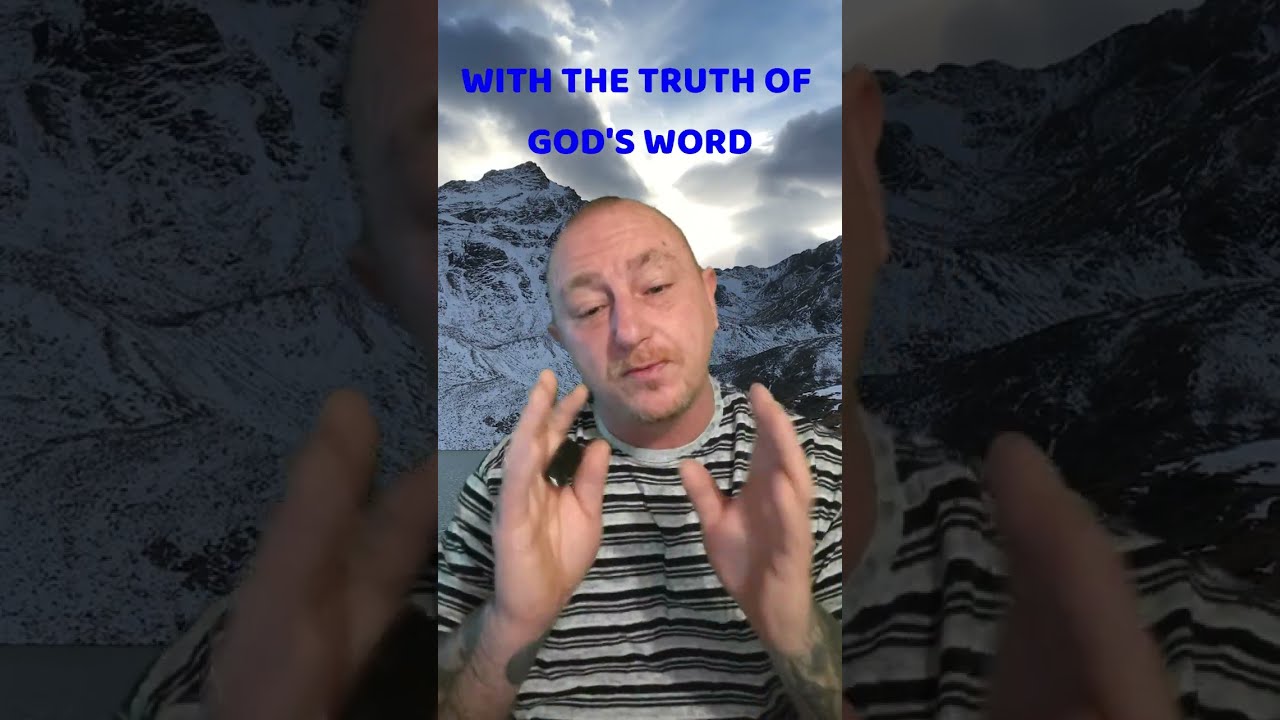The rectangular image consists of three panels, with the left and right panels displaying darkened, close-up angles of the central panel's scene. The primary focus is on an older, mostly bald man with a blonde mustache, short light blonde hair, and blonde eyebrows. He also has a short blonde goatee. The man is engaged in what appears to be a video call, perhaps a social media post or a still from a TikTok video, evidenced by the motion blur on his gesturing hands. He is wearing a short-sleeved white shirt with black stripes and has tattoos on his wrists and forearms. In the center panel, he holds a black object in one hand and seems to be in mid-conversation. The backdrop is a green-screened image featuring a cloudy sky with a hint of sunlight streaming through and a snow-covered mountain peak. Emphasized in dark blue, capital letters above him is the phrase, “WITH THE TRUTH OF GOD'S WORD.”